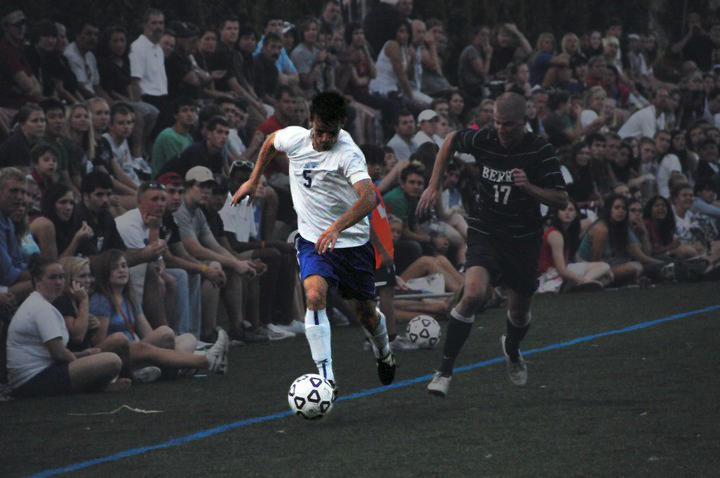In this detailed photo of a European soccer game, two players are competing for control of the ball on a grass field. One player, who has short black hair, is wearing a white T-shirt with the number 5, blue shorts, and white and black socks. This player has the black-and-white soccer ball positioned near his foot. His opponent, who has a buzz cut and wears a black and white striped shirt with the number 17, along with black shorts and black and white socks, is running close by, attempting to intercept or challenge for the ball. The action is taking place near the edge of the field, almost outside the boundary line. Surrounding the players, a vibrant crowd sits on the edge of the field and in the stands, intently watching the game. Among the spectators, a girl with blonde hair is seen talking on her cell phone, seated next to a girl in a white shirt and black shorts, and another girl in a blue shirt. The audience appears engaged and the stands are fairly full, suggesting it could be a night game given the darker ambiance. The image captures the tension and excitement of the match in a horizontal, rectangular frame.